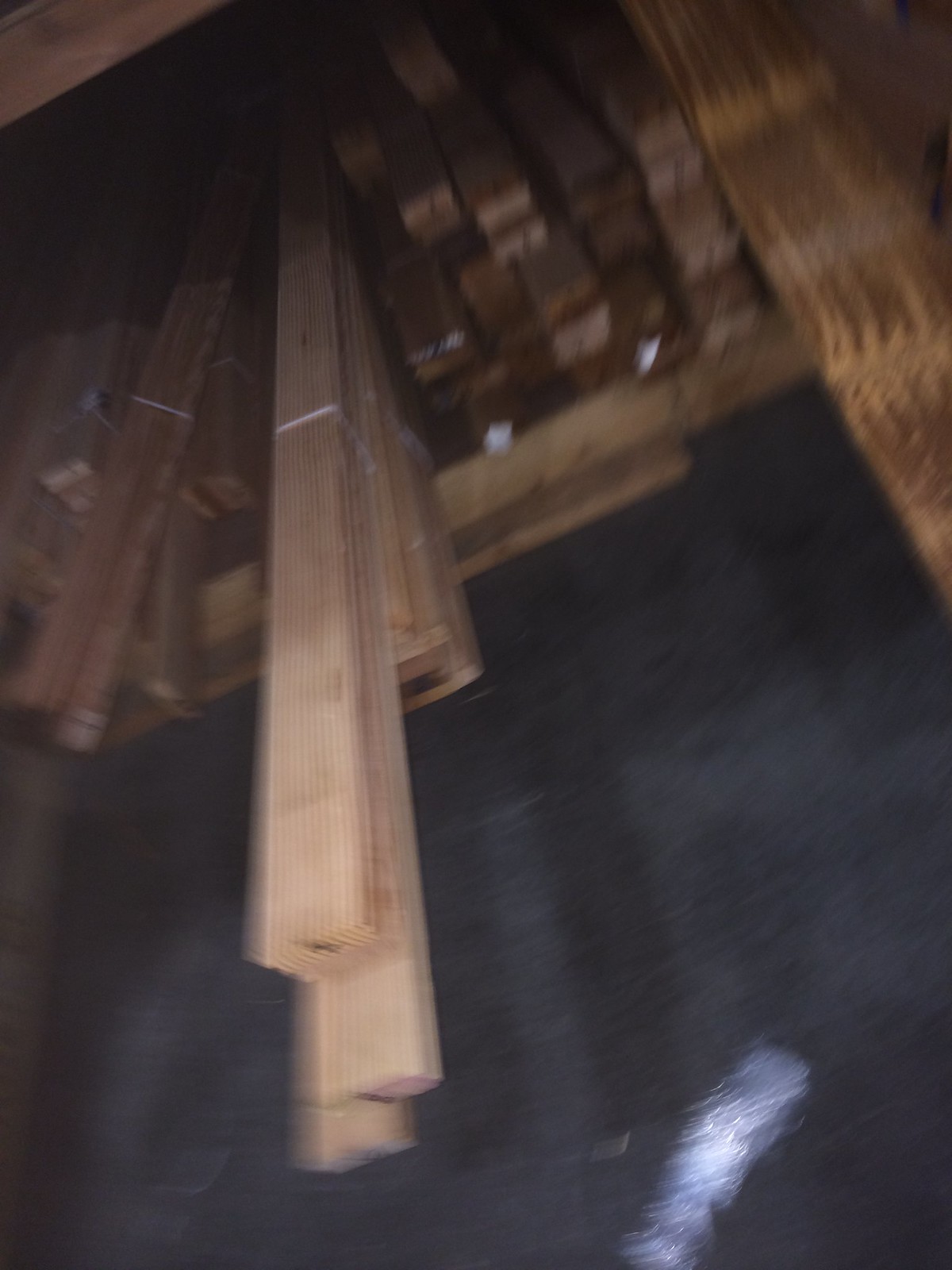The image showcases an indoor scene taken in a large package or box store, depicting an assortment of lumber primarily in the form of 2x4s. The lumber, which ranges in color from natural light browns to darker, possibly pressure-treated hues, is stored on a wooden rack. Some pieces are bundled together with white plastic straps, and the wood appears in various lengths, with some protruding beyond the edge of the rack while others do not. The rack itself sits on a concrete floor that appears dark gray with patches and a light streak, adding to the sense of an industrial setting. The wood piles in the rack are neatly grouped into bundles, and the entire scene is slightly blurred, particularly on the right-hand side where indeterminate dark brown and light brown shapes are visible. The perspective of the photo tilts slightly to the left, showing the upper bin's shelf in the upper left-hand corner and indicating that some lumber pieces have been pulled out for viewing, while others remain back in the lower bin, creating a visually dynamic presentation of the lumber stock.